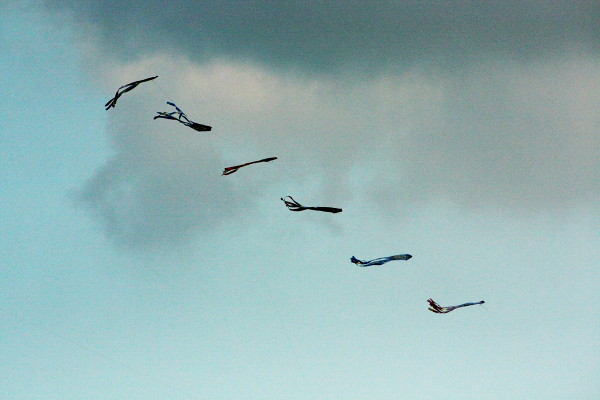The image depicts a serene sky scene, blending shades of mint green to blue, evoking a painted quality. Dominating the center is a wispy cloud formation that extends to the right, resembling soft, fluffy substances. Alongside the clouds, six kites, or kite-like objects, float diagonally from the left to the lower right, with their strings trailing loosely. These strings are unraveled at their ends, with some pointing upwards and others fanning out. The kites vary in color - two appear black, one red, one blue, and another possibly red, though their exact hues are somewhat obscured by the lighting. The sky, a teal backdrop, is sparsely covered by clouds with a dark gray accumulation at the top and a lighter, fluffy cloud towards the center. This thoughtful arrangement of sky and elements captures a peaceful, almost nostalgic aerial view.